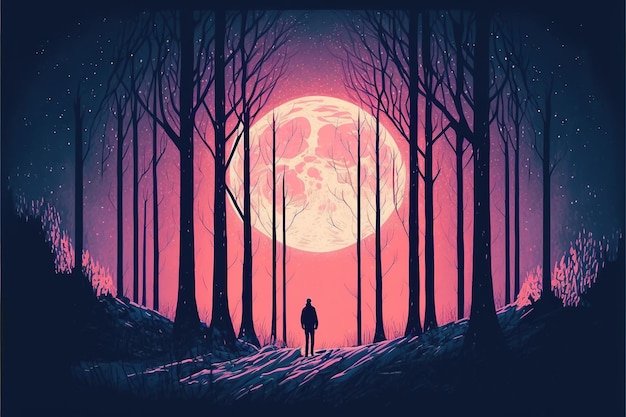In this evocative, digitally illustrated nighttime scene, a vast full moon dominates the center, casting an enchanting pink and purple glow across the sky. The moonlight transitions from a vibrant pink around the moon's edges to a deep purple further out, eventually blending into the dark blue of the star-speckled night. The foreground features the textured silhouette of rocky terrain, enhancing the mystical atmosphere with shades of purple reflecting the moon's light.

Rows of barren, black silhouette trees, their leafless trunks stretching from the ground to the top of the image, frame the scene. In the very center of this ethereal forest, a lone man stands, his figure reduced to a mere shadow. He gazes up at the luminous moon, which is detailed enough to reveal various craters and surface indentations, giving it a lifelike intricacy. The surrounding stars glow softly, embellishing the dark sky and adding to the magical vibe of the scene. The man appears to be standing on a slight incline, further heightening the dramatic perspective as the moonlight casts intricate shadows across the trees.